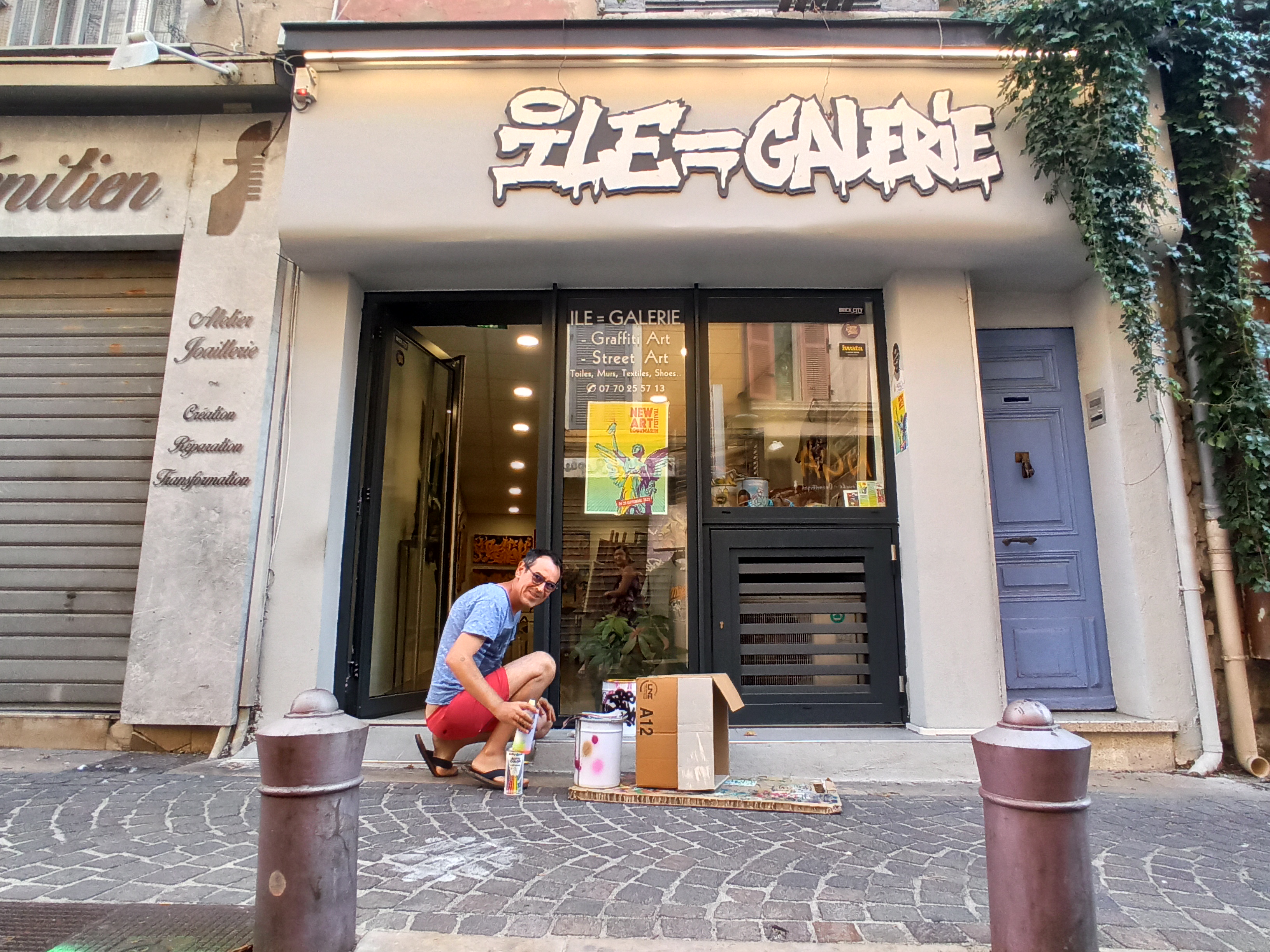The image showcases the front of a gallery named "Le Gallery," located in an urban, metro city setting. A man with dark hair and glasses, wearing a blue shirt and pink shorts, is seen kneeling in front of the store, handling a glass. Beside him are various painting supplies, including a bucket and a cardboard box. The sidewalk, made of stone and brick tiles, features two metal posts with half-circle tops in the foreground. The gallery windows display the phrases "graffiti art" and "street art" and have a poster visible. A tiny blue door is situated to the right of the storefront, accompanied by green ivy hanging down from the building. On the left, another business with a metal garage door is partially visible.